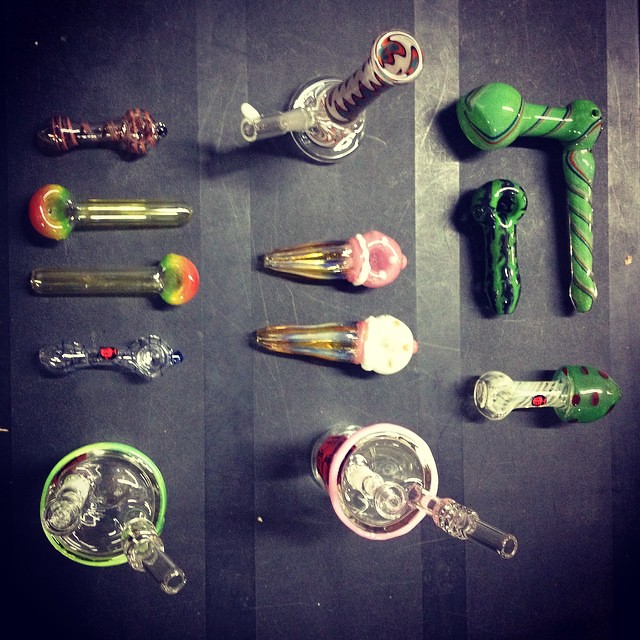The image features a top-down view of a collection of 13 colorful, hand-blown glass pipes, likely used for smoking marijuana, meticulously arranged on a black, scratched surface, which might be a floor or a counter. The pipes exhibit a variety of vibrant colors and designs. Several pipes are transparent or have intricate patterns, including green with black and red stripes, and some are themed—three pipes resemble mushrooms with green and red spots, while two are crafted to look like ice cream cones. Additionally, there are pipes with distinct rainbow hues, evoking a Bob Marley aesthetic. The arrangement is color-coordinated with clusters of green, pink, and multi-colored pieces, reflecting a playful and artistic display, typical of a setting where smoking accessories are part of the person’s lifestyle.